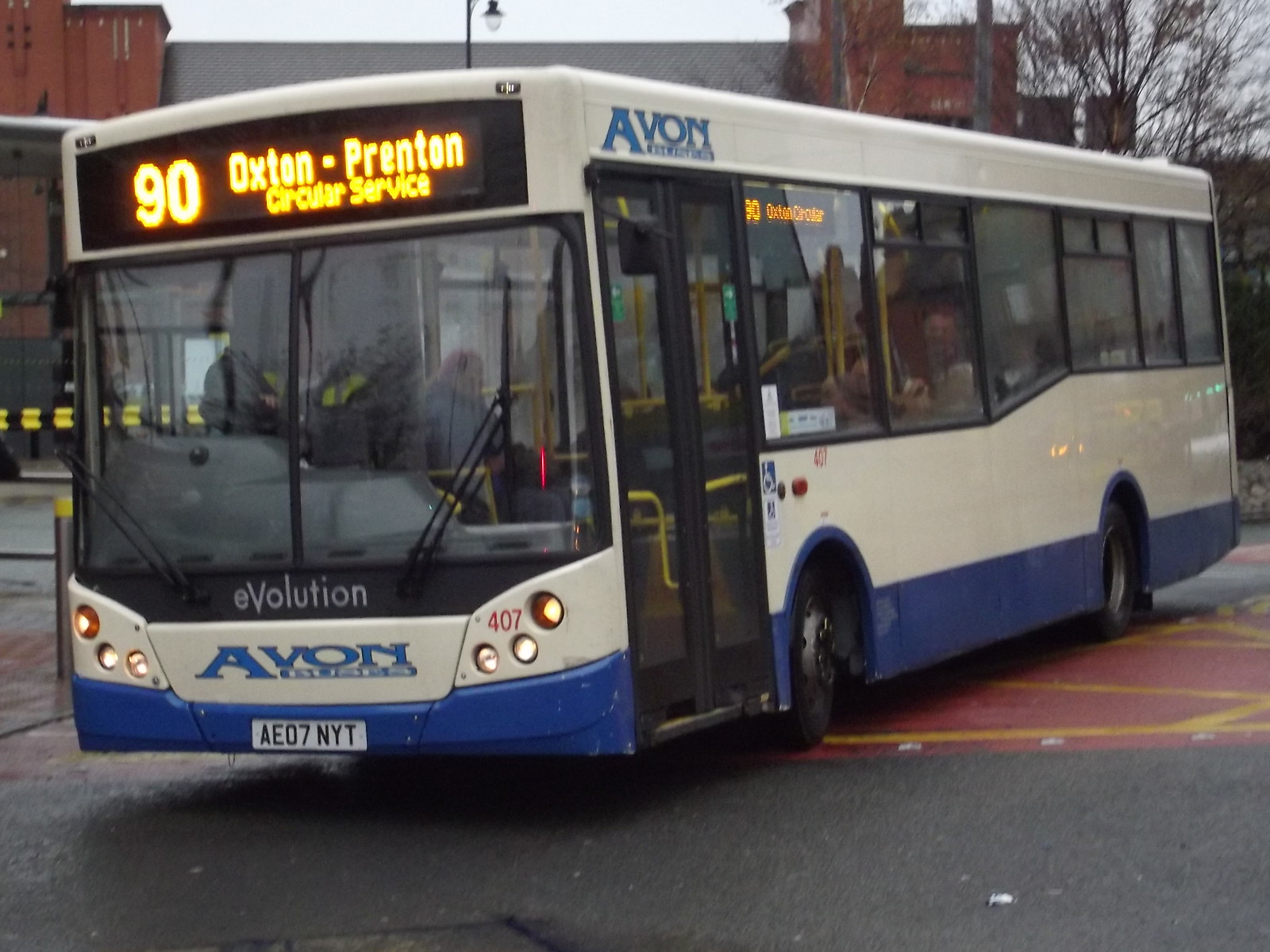The image depicts a city bus with a blue bottom and white top, prominently featuring "Avon" in blue font on both the front and just above the door on the side. The front license plate reads AEO7NYT, and the word "Evolution" is displayed in white under the windshield. The bus's LED screen sign indicates "90 Oxton-Prenton Circular Service." The front of the bus includes large, flat glass windows, and the bus has headlights on. There are people visible seated inside through the side windows. In the background, various buildings can be seen, including a structure with a gray roof flanked by rusty red buildings. The sky is overcast, adding to the scene's detail. The bus appears to either be parked or making a turn on a city street, with some lines visible underneath it, hinting at its position.